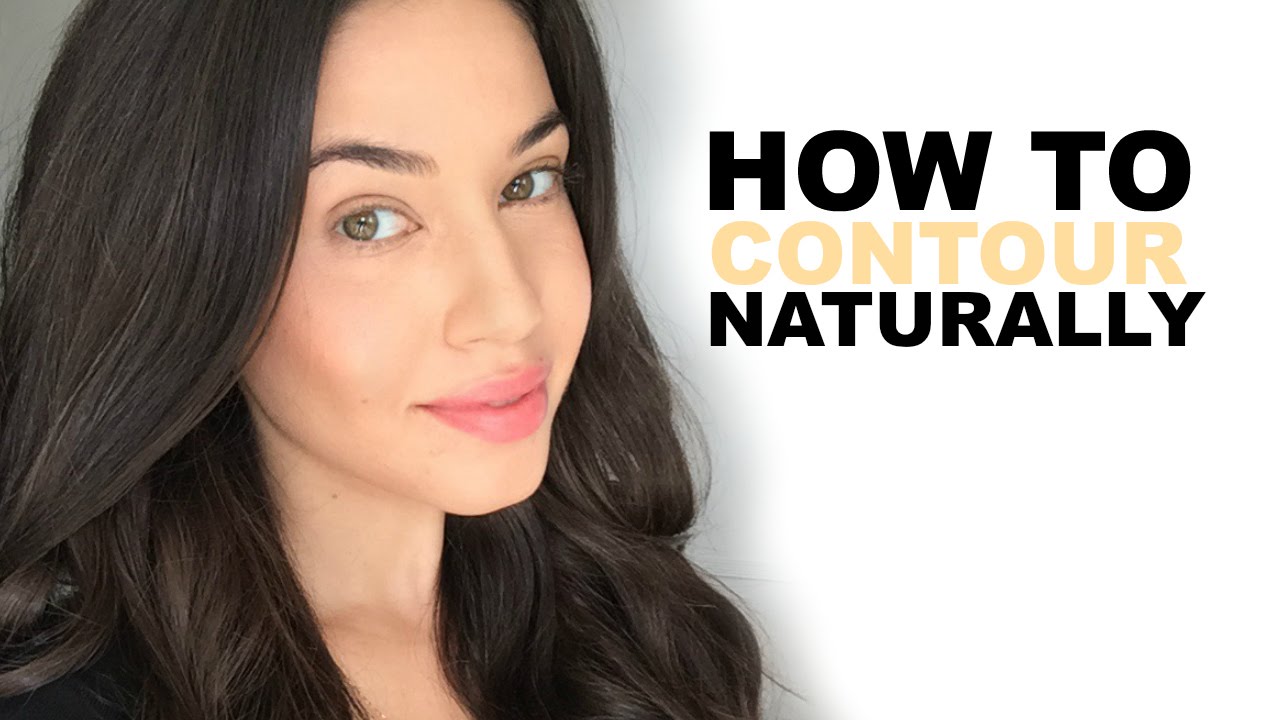This appears to be a cropped image likely derived from a YouTube video or thumbnail, presenting a tutorial on "How to Contour Naturally." On the right side of the image, over a white background, bold black text reads "How to Naturally," with the word "contour" highlighted in a yellowish-tan color to emphasize the tutorial's focus. To the left, a close-up of a woman's face dominates the frame. Her complexion suggests she is Caucasian, and she has thick, long, dark brown hair parted in the middle, cascading past her shoulders and obscuring most of her black blouse. She gazes slightly leftward with her head tilted in that direction, her lips forming a subtle, close-mouthed smile. The woman has captivating green or hazel eyes and full, pink lips that hint at light makeup, enhancing her natural beauty. The contrast between the white text background and the gray backdrop behind her head, especially noticeable in the upper left corner, adds depth to the image.